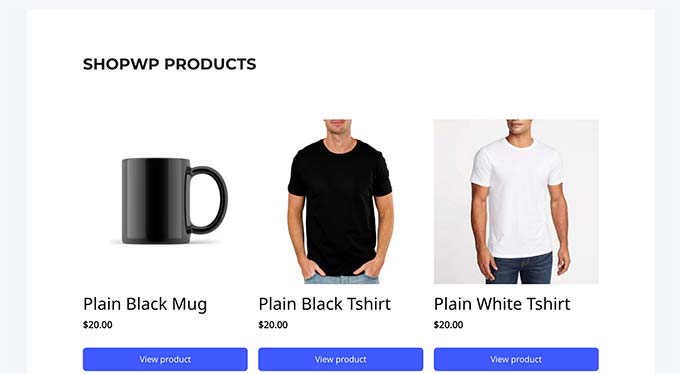This image showcases a selection of "SHOP WP PRODUCTS," prominently displayed in bold, black, all-caps font at the top. The background consists of a white box overlaying a barely-visible gray box, with the edges peeking out from the top, left, and right sides.

Within the white box, three items are neatly arranged in a horizontal line:

1. On the far left is an image of a plain black mug, positioned with its handle on the right side. Below the mug, the label reads "Plain Black Mug." The price is listed as $20, and there's a "View Product" button underneath the price.

2. In the center, there's a plain black t-shirt. Its straightforward design is highlighted by a label that reads "Plain Black T-Shirt," priced at $20, with a "View Product" button found below the price.

3. On the right, a plain white t-shirt completes the lineup. The label beneath it reads "Plain White T-Shirt," also priced at $20, accompanied by a "View Product" button below the price.

The structured layout and clear labeling ensure easy navigation and a pleasant visual experience for potential customers.